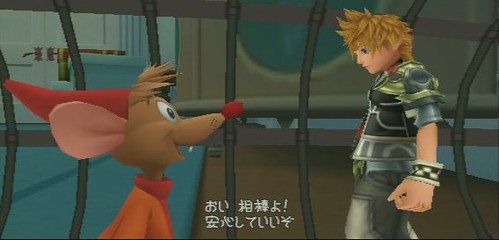This detailed screenshot originates from one of the Kingdom Hearts games, though the specific installment is not immediately clear. The scene features a notable interaction between a mouse character from Cinderella and the protagonist of Kingdom Hearts. The setting appears to be the interior of a ship or possibly a submarine, given the oceanic elements visible. In the background, a porthole reveals an underwater scene with vessels, emphasizing the maritime or subaqueous environment.

Foregrounded in this image are the two characters. On the left, the mouse, dressed in a red hat, an orange jacket, and a red shirt, is seen mid-conversation with his mouth open, facing right. Opposite him, the Kingdom Hearts protagonist, distinguished by his yellow hair and a distinctive futuristic ensemble that includes a jacket, wrist bracelet, and pants, faces left. They both seem to be enclosed within a cage-like structure, suggesting they might be trapped or imprisoned in an underwater jail.

Japanese text in white overlays this animated cutscene, indicating that it is a dialogue sequence within the game, contributing to the narrative progression typical of Kingdom Hearts titles.